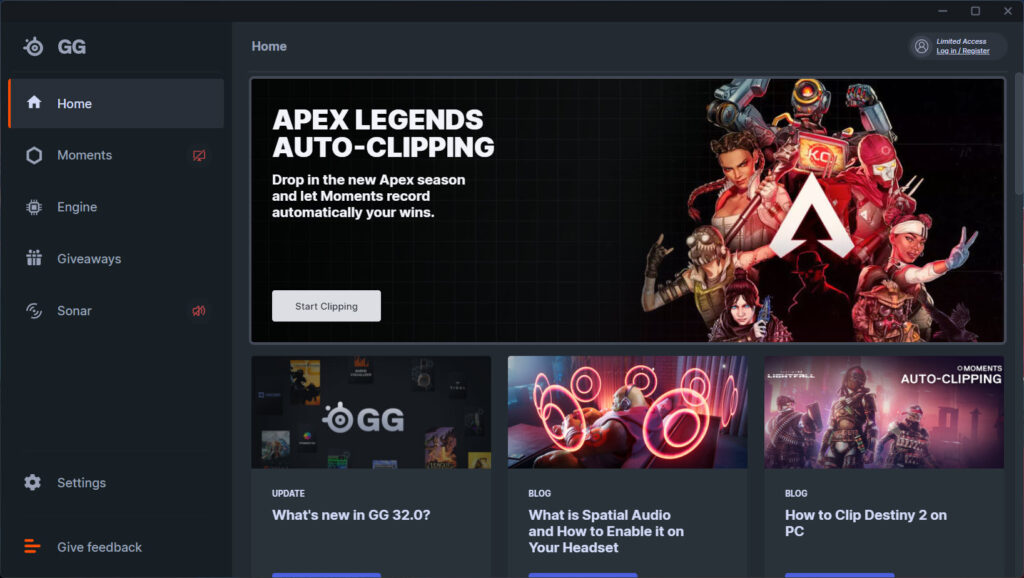Screenshot description:

The screenshot captures a specific view of a gaming app's website. Dominating the top left corner, an icon marked with "GG" stands out against a gray backdrop. A vertical menu list is prominently featured beneath this icon, comprising the following items: Home, Moments, Engine, Giveaways, Sonar, Settings, and Give Feedback. The "Home" option is distinctly highlighted by a red banner.

Each menu item is accompanied by relevant symbols: Moments has a circular icon, Engine is paired with a gear icon, Giveaways boasts a gift box symbol, Sonar is denoted by a small sound device icon, Settings share the gear symbol with Engine, and Give Feedback is marked by three uneven lines in red. On the right-hand side of the Moments, Engine, and Sonar items, there's a red icon suggesting a sharing feature.

On the right side of the screen, a section labeled "Home" contains a notable central image. This section promotes "Apex Legends Auto Clipping," encouraging users to launch the new Apex season and automatically record their victories through the Moments feature. Below this promotional text is a white button with black text labeled "Start Clipping." Adjacent to this promotional content, a collection of character icons, including a robot, a steampunk persona, and a warrior, adds visual engagement.